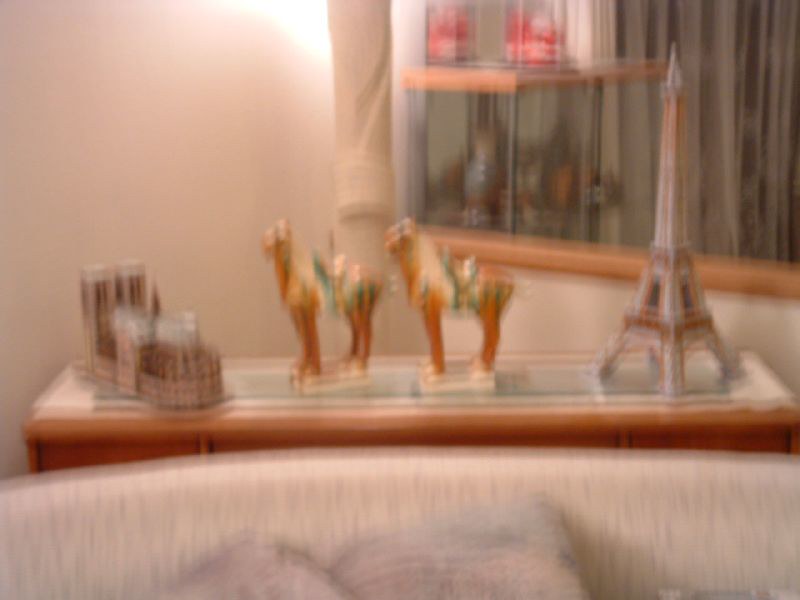The photograph depicts a slightly blurry yet cozy living space with a focus on a white sofa with pastel-colored cushions in the foreground, featuring shades of pink, blue, and white. Behind the sofa, a medium brown wooden console table, taller than the sofa itself, is adorned with a long white cloth and a piece of glass running across it. On top of this glass-covered surface is a collection of decorative sculptures, including two ceramic horses styled after the Tang dynasty in light brown hues, positioned at the center. To the right of these horses stands a detailed model of the Eiffel Tower in gray and brown colors, while to the left is a model of a French cathedral, possibly Notre Dame, characterized by its intricate towers and architectural details. In the background, a partly visible glass cabinet contains indistinguishable items, complemented by a warm red and brown color scheme. Additional elements include a white wall with uplighting in the corner, a white privacy drape, and a low dividing wall.